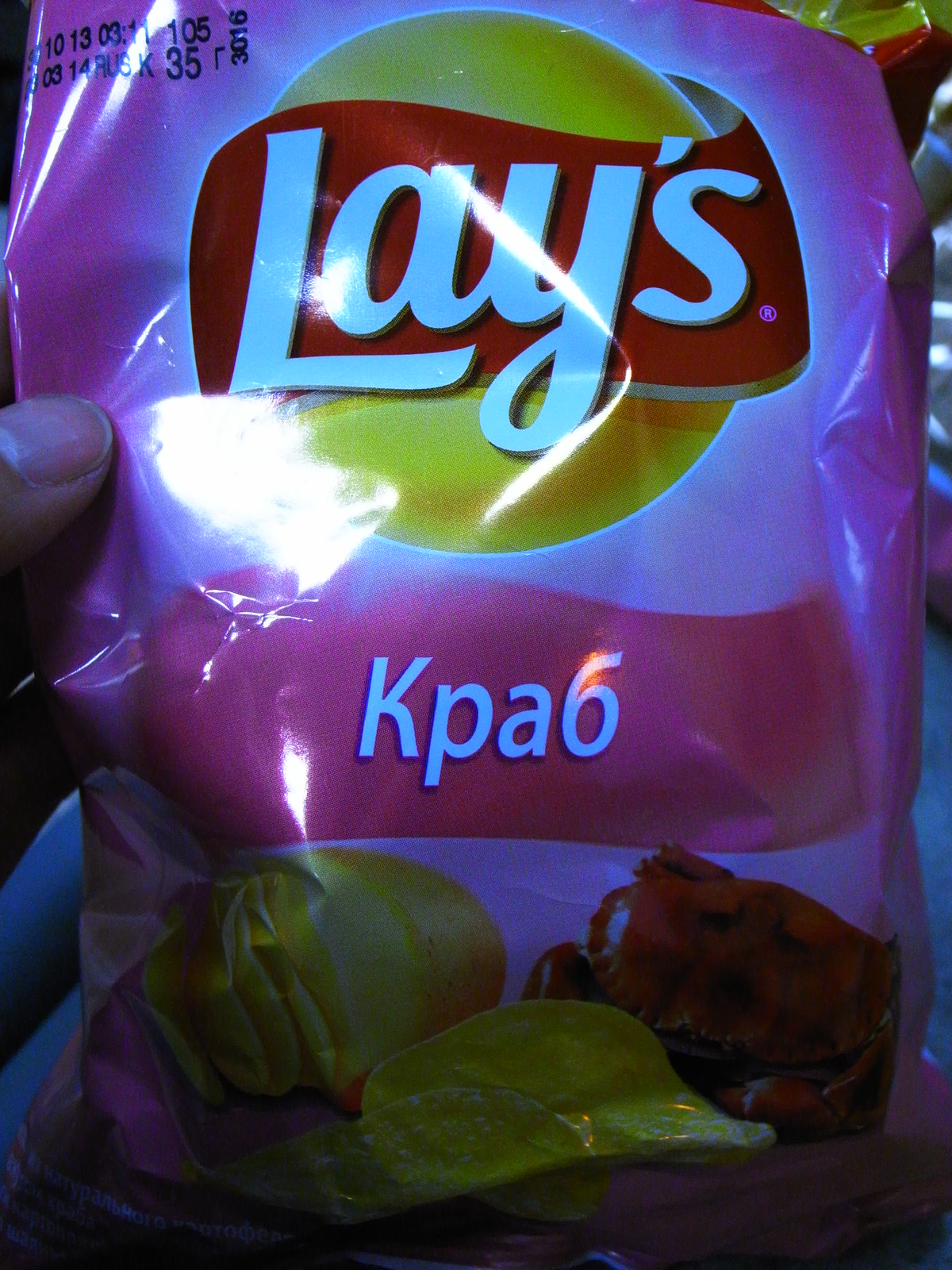This is a close-up image of a brightly colored, tall, and shiny bag of Lay's potato chips in portrait mode. The bag is predominantly light pink with the iconic Lay's logo prominently displayed at the center. The Lay's logo consists of "Lay's" written in white font over a red banner with a yellow circle backdrop. Directly beneath the Lay's logo is a pink banner that reads "KPA6," indicating the flavor, which appears to be prawn cocktail or a similar flavor. The bottom portion of the bag features images of yellow potato chips and a red crab-like blob. The lighting in the photo is not optimal, casting a notable brightness spot just under the 'L' of the Lay's logo and leaving the bottom of the bag quite dark. The use-by date and other numeric details, such as C1013, 0311, 105, 0314, RUSK35, and 306, are printed in black at the top left corner. A thumb and part of a finger can be seen holding the bag from the left side, with no other notable elements in the background.